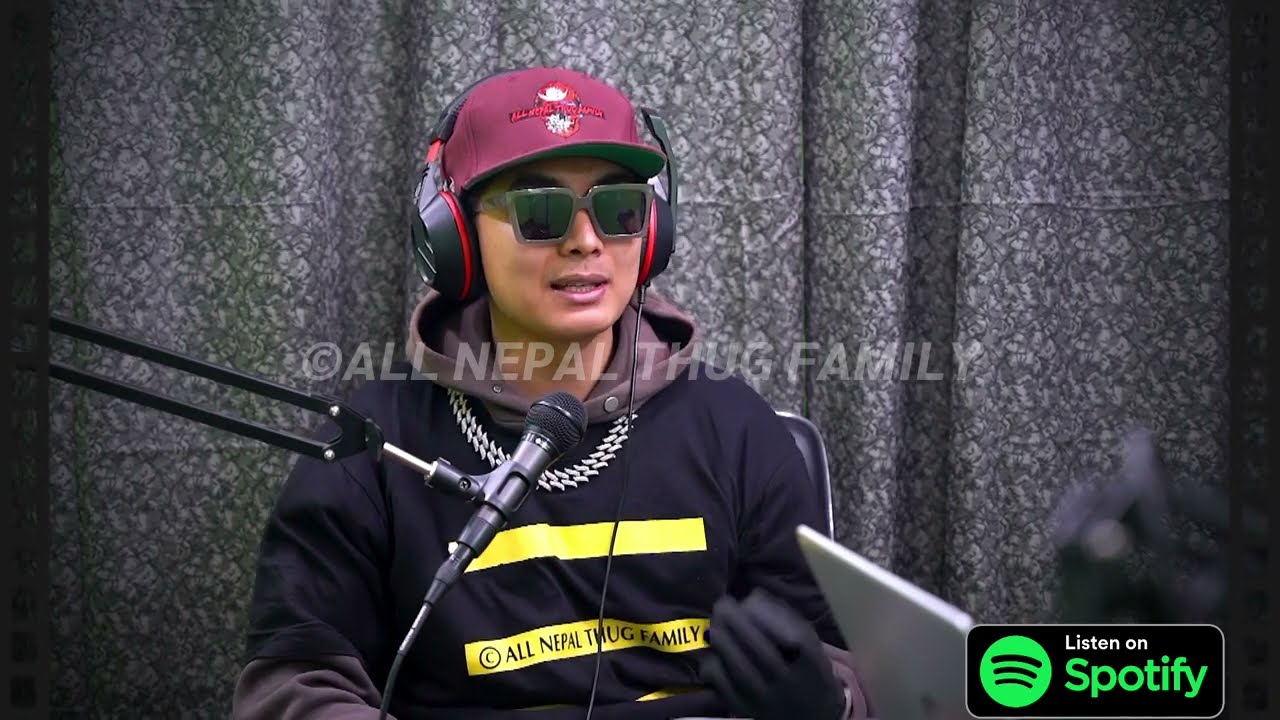In this detailed photograph taken in an indoor setting, a man is prominently seated at the center. He is wearing a red baseball cap adorned with a white design and dark pink wording, along with black square-shaped sunglasses featuring gray rims. Over his ears, he sports black headphones with red trim, and he appears to be speaking into a standing hand-free microphone situated in front of him. The man is clad in a black T-shirt with two yellow horizontal stripes across the chest, displaying the words "All Leopard Flock Family." Behind him, a gray curtain with white patterns serves as the backdrop, adding texture to the scene. The bottom right corner of the image features a logo, a circular green Spotify icon with three black lines, accompanied by the text "Listen on Spotify."